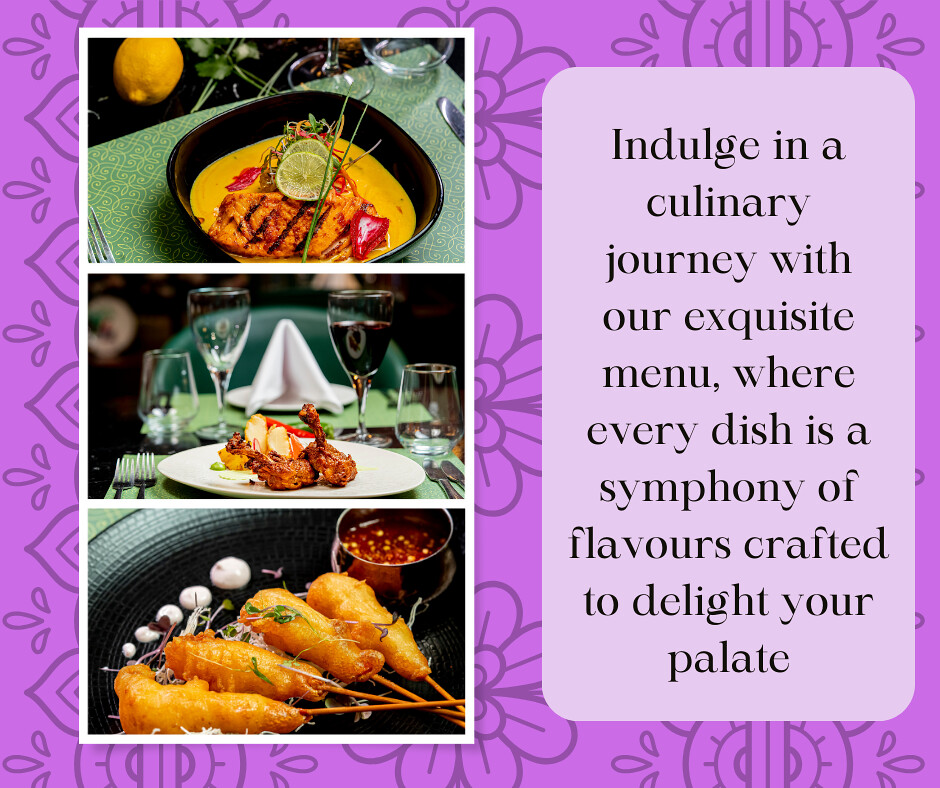The image showcases a visually striking poster featuring three distinct dishes against a light purple background adorned with intricate floral illustrations. On the left side, three photos are vertically stacked and outlined in white, each presenting a delectable dish.

At the top, the first photo displays a sumptuous bowl with a thick orange puree, topped with a grilled chicken breast adorned with lime slices, fresh herbs, and pepper, all set on a vibrant green tablecloth alongside wine glasses and a lemon.

The middle photo presents a pair of well-seasoned chicken wings, elegantly garnished and accompanied by two forks on the left and two knives on the right. Behind the plate, an assortment of glasses and a meticulously folded white napkin complete the table setting.

The bottom photo features what appears to be sweet and sour chicken, coated in a light breading. The dish includes four corn dog-like pieces served with a peppery dipping sauce in a silver container, garnished with white cream dots.

To the right of these enticing images, a message in elegant font reads: "Indulge in a culinary journey with our exquisite menu, where every dish is a symphony of flavors crafted to delight your palate."